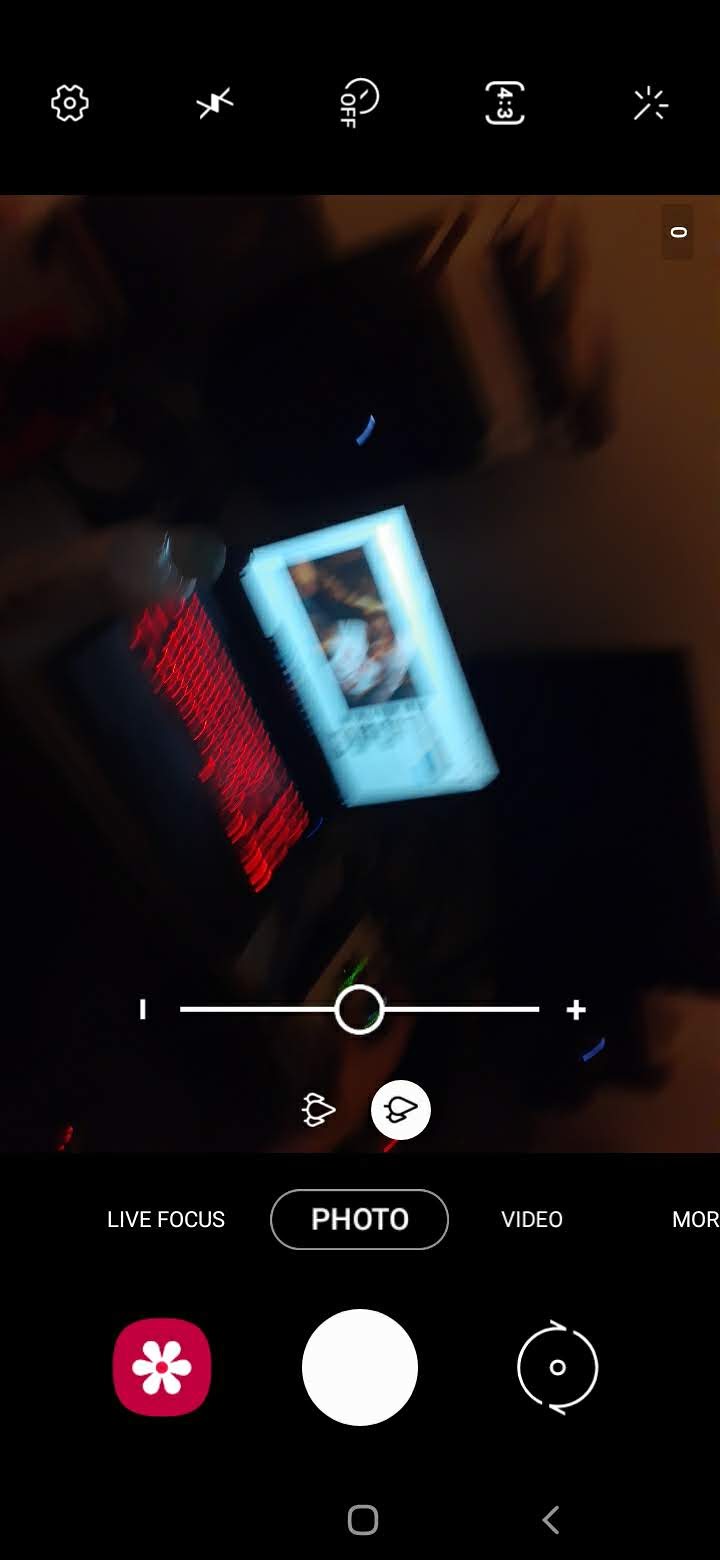This image depicts a smartphone screen with a detailed interface visible. At the top, there are five icons positioned sideways. Starting from the left, the labels beneath the icons read sequentially as: "Live Focus," "Photo," and "Video." Directly below these icons, there is a square artwork with rounded corners, featuring a delicate white flower centered within it. To the right of this artwork, a prominent round white circle is visible, likely a button or interface element. Further to the right, another round circle can be seen, continuing the layout of the screen's elements. The image captures the intricacies of the phone interface, highlighting various features and icons available for user interaction.